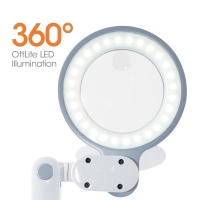This image depicts a circular LED light, designed for camera work, particularly useful for on-camera appearances. The light is prominently showcased with an outer frame in grey, encompassing an array of small LED bulbs arranged in a circular pattern. In the center of this circular array, there might be a larger light source, though it is somewhat indistinct. The text "360 degrees" is displayed in bold orange font at the top of the image, indicating the light's comprehensive, all-around illumination capability. Below this, the phrase "off light LED illumination" is written, describing the nature of the lighting.

The LED circle light is affixed to a white handle, which is detailed with grey accents that could be bolts, plugs, or buttons, adding functional elements to its design. The entire assembly appears sleek and professional, suggesting it is engineered for optimal lighting without being overly harsh. The background of the image is stark white, ensuring that the light and its details are the focal point without any distractions. This product likely aims to provide balanced, soft illumination, ideal for ensuring clear and comfortable visibility of a subject's face during camera work.